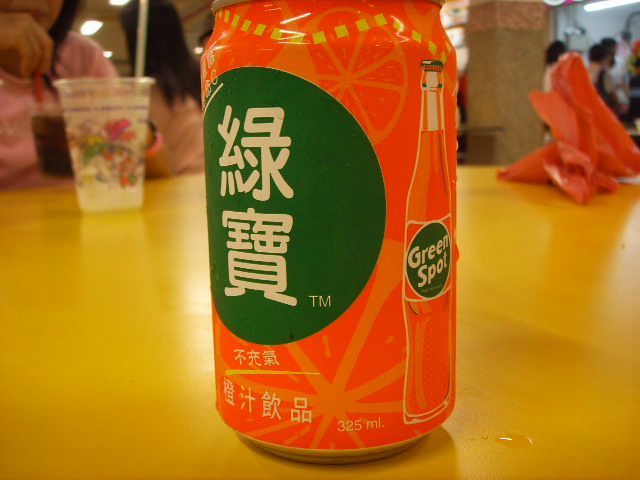In this detailed photograph, we are placed within what appears to be a bustling cafeteria or restaurant, possibly within a shopping mall characterized by overhead lighting and a ceiling peeking into view. The majority of the image is dominated by a yellow-brown wooden table, which plays host to various objects and figures, illuminated by differently lit spots that cast distinct shadows.

At the center of the image is an aluminum can of soda, predominantly orange in color, with intricate orange designs subtly embedded in the background. The can features a prominent green circle containing white characters from a foreign language along with the initials TM. A dotted yellow line cascades from the top of the can. On the right side, the can displays an illustration of a vintage-style soda bottle capped like an old-fashioned Coke bottle, featuring a green circle with "Green Spot" inscribed in white text. The can is marked with "325 ml" at the bottom and is topped off with a small droplet of water visible at the bottom right corner.

To the left of this can, a person in a pink top with long black hair, not fully facing the camera, is discernible. They are sipping from a dark brown liquid. Situated in front of them is a clear plastic cup with red, white, and green decorations, an inserted white straw, and a transparent liquid inside. Additionally, there is a person partially visible in the upper left-hand corner of the image, seen holding a red fork inside a drink. There is also an orange shopping bag and a piece of orange paper partially seen at the edges of the table.

In the background, against a white wall, people are either ordering or socializing, contributing to the lively ambiance. The scene is partially obstructed by a tan concrete post, suggesting additional ordering counters behind it, indicative of a typical shopping mall layout.

Overall, this photograph captures a vivid and bustling moment, marked by the ordinary yet intricate details of a shared public space.